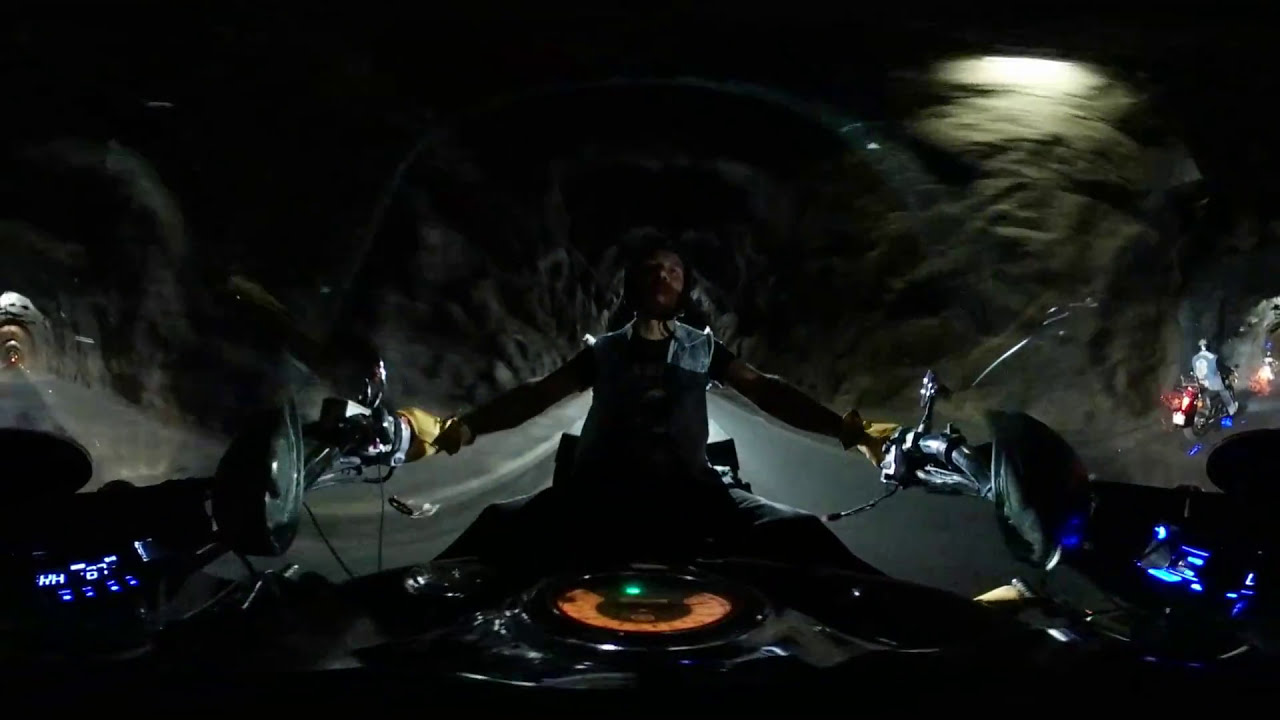The image portrays a bearded man in dark clothing, lying down as if reaching for motorcycle handlebars, suggesting he's riding a bike. The setting appears to be nighttime on a street, illuminated by backlighting with a blurred streetlight visible in the upper right quadrant. A crashed, gray-colored car seems to surround him, indicating a potential accident scene. Visible elements include an orange circle with a green dot beneath him and yellow objects near his hands. The image, likely distorted by a 360-degree lens, has a predominantly blackish-gray background with light reflections on the right, and contains digital signage suggesting a graphical or video game-like design.